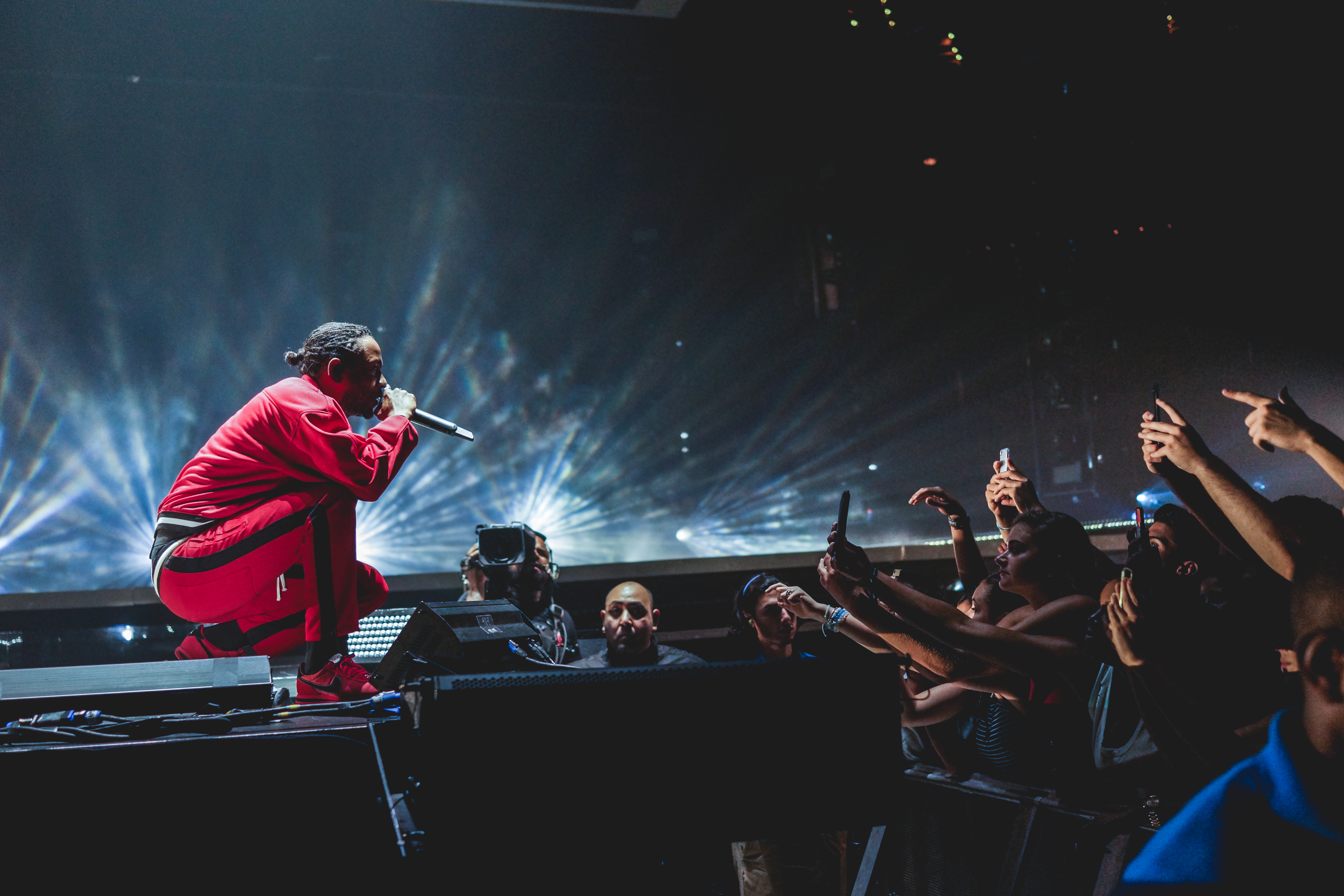The image captures a dynamic scene of Kendrick Lamar performing at a concert. Positioned in the left foreground, Kendrick, a younger to middle-aged black man, crouches low, demonstrating impressive flexibility. He sports a distinctive man bun and is dressed in an eye-catching red athletic jumpsuit with black stripes down the sides of his legs and additional black accents at the waist. In his right hand, he clutches a wireless microphone, bringing it close to his mouth as he intimately engages with the roaring crowd.

On the right side of the image, a sea of enthusiastic fans can be seen, with numerous hands reaching into the air, some holding cell phones to capture the moment. Among the audience, a few men with stern expressions, likely bodyguards, stand between Kendrick and the fans, ensuring his safety.

The background is illuminated with starburst-like stage lighting, creating a dramatic effect against the predominantly dark backdrop. Multiple light sources contribute to the visual spectacle, adding to the energy and intensity of Kendrick's performance. The stage atmosphere is bustling with vibrant, synchronized lights and the palpable excitement of the concert-goers.